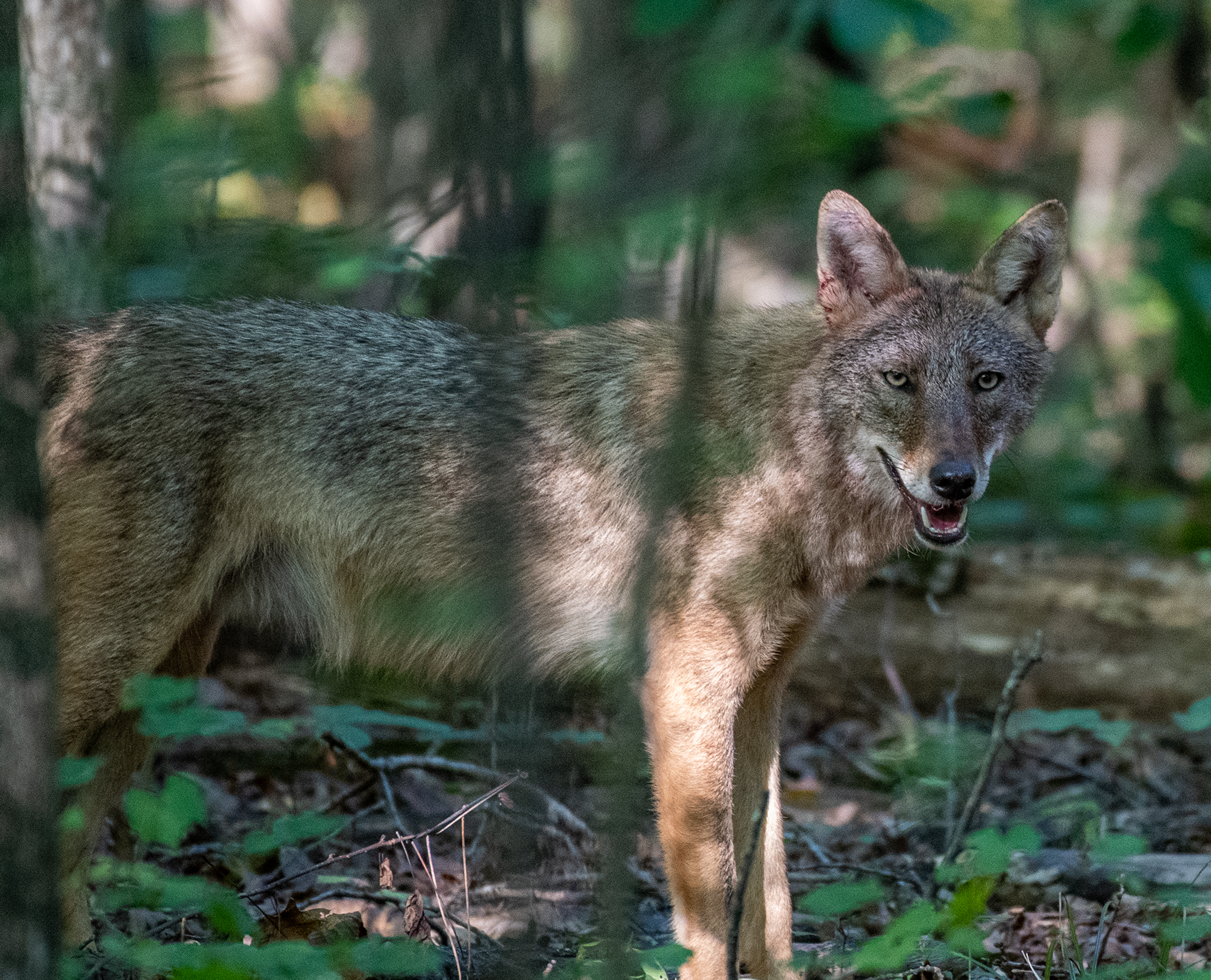In this evocative photograph, the focal point is a lone, malnourished wolf standing alert on a forest floor strewn with green leaves and a tangle of brown twigs. The wolf, with its gaunt frame and haggard coat that is black near the top and fades to white near the bottom, exudes a quiet desperation. Its tannish legs add to its emaciated appearance. The animal's head, with its mouth open to reveal sharp, white canines, is turned towards the right side of the image, while its alert, erect ears and wary eyes suggest a mix of caution and fatigue. The tail, positioned towards the left, and the compelling, powerful gaze add a layer of majesty to the otherwise fragile creature. In the blurred background, the mixture of green foliage and brown branches hints at a dense, possibly jungle-like forest, accentuating the wolf’s stark presence against the natural backdrop. The scene is both mesmerizing and unsettling, capturing the raw survival instinct of the wild.